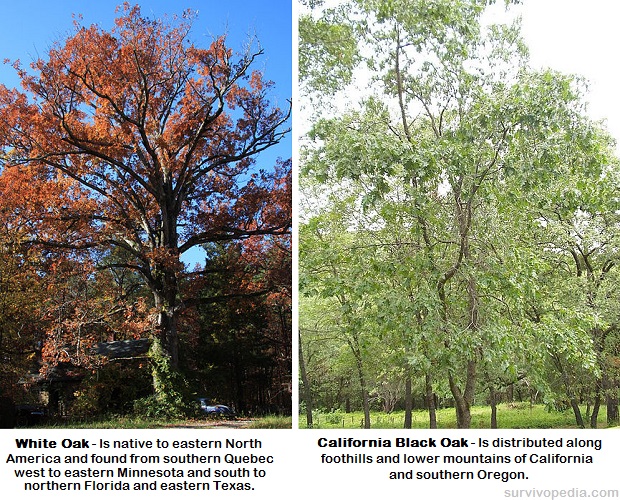The image presents a side-by-side comparison of two types of oak trees. The left photo features a tall California oak with thick branches and red leaves, likely captured during fall, set against a backdrop of other changing trees, blue skies, green grass, and a brown trail. The accompanying text explains that the white oak is native to eastern North America, ranging from southern Quebec to eastern Minnesota, and extending south to northern Florida and eastern Texas. Conversely, the right photo depicts a California black oak with thin branches and vibrant green leaves, standing against a white sky and grassy field. The text below this image notes that the California black oak is commonly found in the foothills and lower mountains of California and southern Oregon. The information in both images is framed with black text on a white background and sourced from Cervivopedia.com.